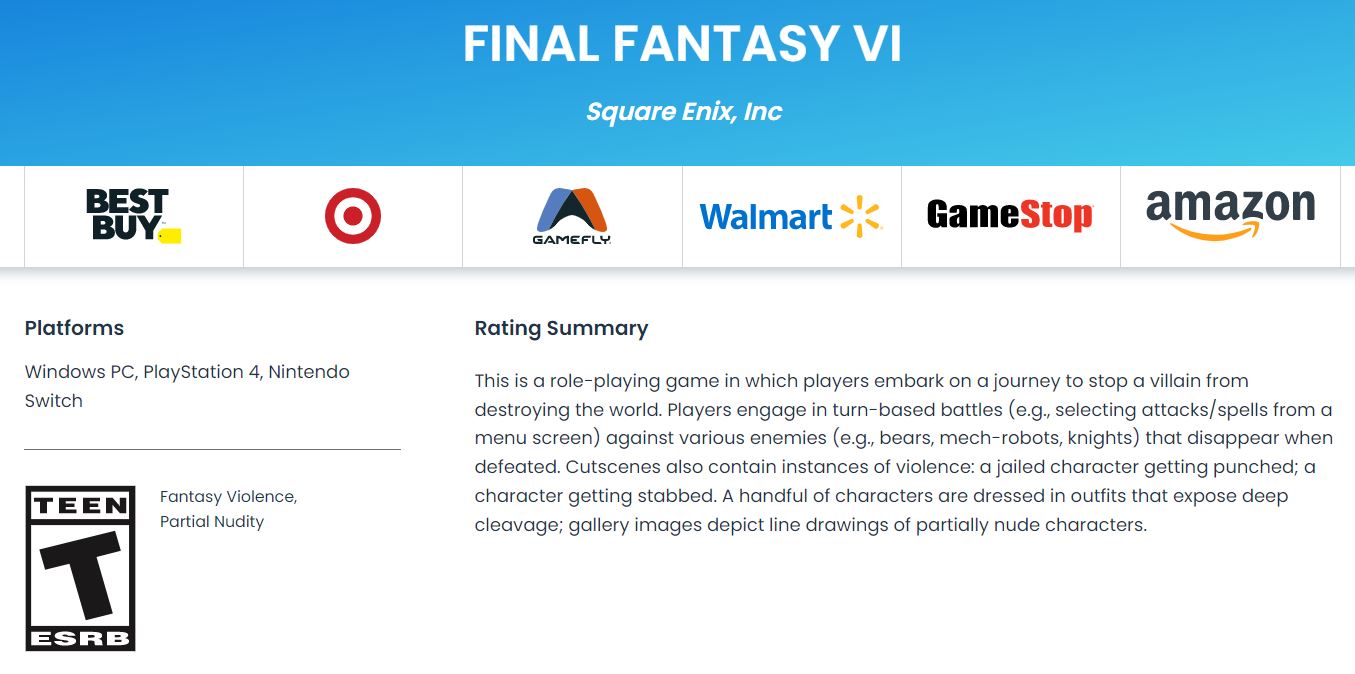The image features a predominantly white background with several key elements:

- At the top, there is a blue box with white text that reads, "Final Fantasy 6" and "Square Enix Incorporated."
- Below this, there are logos for several retailers: 
  - Best Buy (featuring a yellow tag)
  - Target (depicted with its iconic red bullseye)
  - Gamefly (in blue, black, and orange)
  - Walmart (in blue, with a small yellow sunburst)
  - GameStop (in black and red)
  - Amazon (in gray, with its signature yellow swoosh arrow)

- A horizontal blue line separates these logos from the next section.
- The platforms listed include Windows PC, PlayStation 4, and Nintendo Switch.

- Further down, there is another dividing line followed by an ESRB rating box:
  - The box contains a large "T" indicating the game is rated "Teen."
  - It specifies content descriptors: "Fantasy Violence" and "Partial Nudity."
  - The rating summary provides detailed context: It describes the game as a role-playing game where players embark on a mission to prevent a villain from destroying the world. Players engage in turn-based combat, selecting attack spells from a menu to battle various foes, including bears, mech robots, and knights who vanish upon defeat. 
  - It mentions that the game contains cut scenes with violence, such as a character being punched while jailed and another being stabbed. Additionally, some characters wear outfits that reveal deep cleavage, and gallery images include partially nude characters.

The overall composition provides an extensive overview of the game's rating, content, and availability across various retailers and platforms.